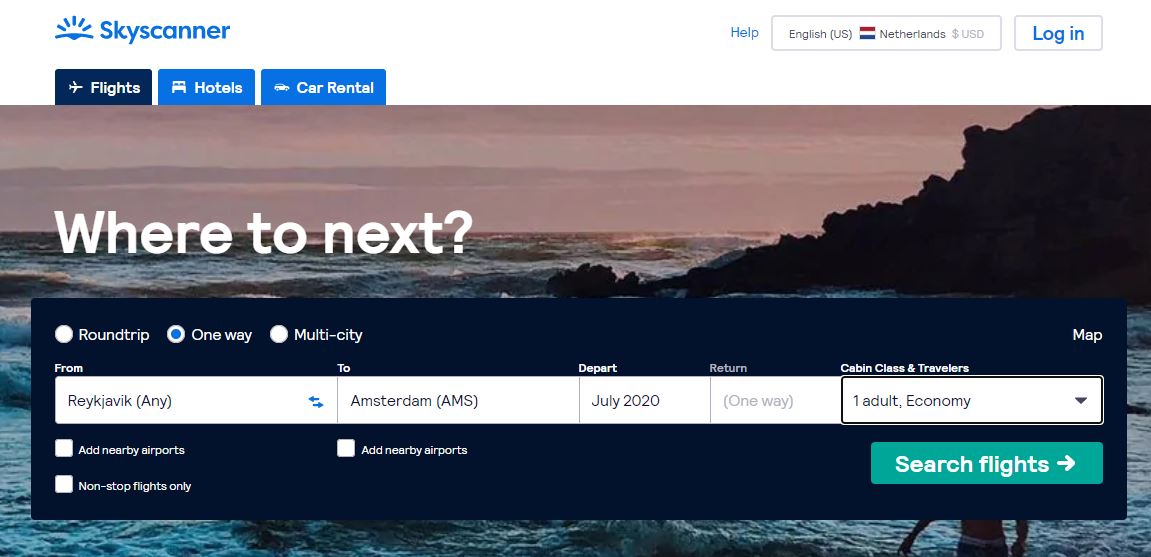This image captures a screenshot of the Skyscanner website. In the top left corner, the Skyscanner logo features the blue text "Skyscanner" alongside a minimalistic blue graphic depicting the sun rising over a hill. Positioned in the top right corner of the site, there are various options including a hyperlink titled "Help," a selectable language and nationality bar displaying "English (US)" and "Netherlands," and a USD currency symbol. Additionally, a blue "Login" button is present.

The main section of the webpage is designed for booking travel arrangements, specifically flights. At the very top, there are three tabs labeled "Flights," "Hotels," and "Car Rental," each accompanied by corresponding icons. The active tab is "Flights." Beneath these tabs appears a large image banner showcasing a scenic coastline with a beach, characterized by a person standing in the bottom right corner. The sky features purple hues, suggesting a sunset atmosphere. Overlaying this image is text that reads "Where to next?"

Below this inspirational prompt is a dark blue card containing fields for flight search details. These include options for a round trip, one-way, or multi-city journey. Additional fields prompt users to specify departure and return locations, dates, cabin class, and the number of travelers. Accompanying these fields are checkboxes for further specifications. A prominent green "Search flights" button is located at the bottom of the card, ready for user interaction.